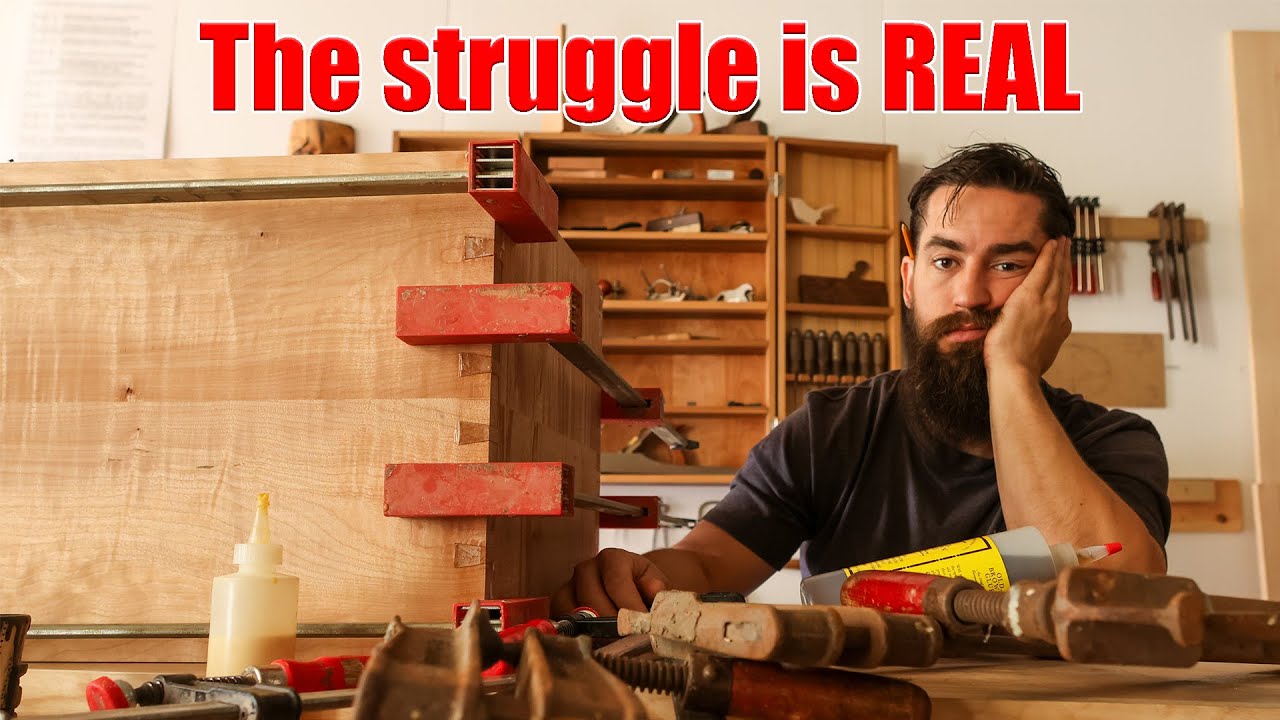In the photograph, a white man with short brown hair and a long, bushy beard with a pencil tucked behind his ear sits in a woodworking shop looking discouraged, propping his head up with his right hand as he stares into the camera. In front of him is a cluttered workbench scattered with various woodworking tools, including clamps, saws, and several bottles of wood glue, one of which is tilted over. To his left, there's a partially constructed wooden shelf. The background features additional woodworking items, tools hanging on the walls, and open cabinets. Above his head, in large, bold red letters, the phrase "The struggle is real" is written, with "real" in all caps.